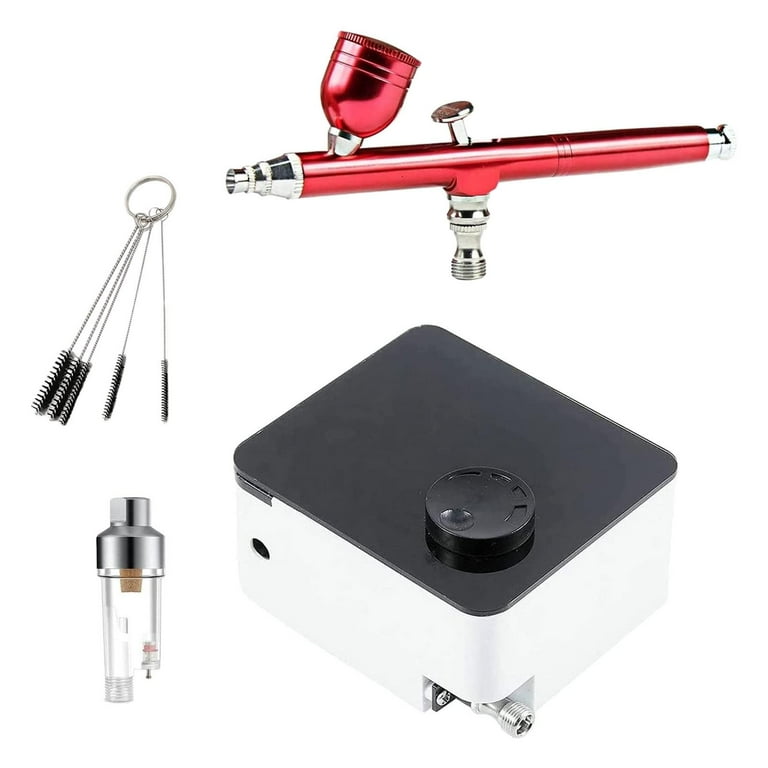This photo showcases a detailed cutout of an airbrush set on a white background. The set features a metallic airbrush tool with a distinct pink metal, almost candy-red color. The airbrush has a reflective, painted finish with a silver knob at the bottom, a silver button on top, and a silver spray nozzle. Attached to the top of the airbrush is a small bowl designed to hold paint. To the left, there are cleaning tools consisting of small metal brushes, and in the bottom corner, a glass case likely intended for storing paint or cleaning fluid. The airbrush connects to a square-shaped pump, which has rounded edges and a black dial on top to control the spray strength. The pump has a metallic nozzle on one corner and a white underside. This set is versatile, suitable for tasks such as makeup application, artistic projects, and other small-scale endeavors.